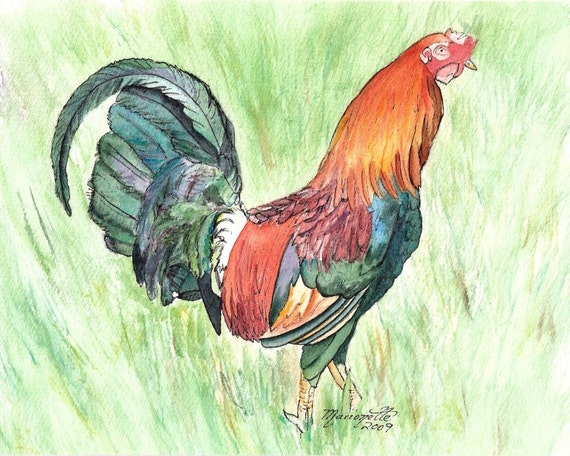This is a meticulously detailed pencil drawing of a rooster, facing to the right against a lightly textured grassy background. The artist's signature adorns the bottom of the artwork. The rooster boasts a striking reddish neck and a vibrant red bill, with a sharp, pointy beak. Its feathers exhibit a rich blend of bluish and reddish hues, rendered with intricate texture. The lower part of the wing features shades of orange, while the rooster’s long, fluffy tail is accentuated by one specific feather that protrudes, curving slightly above and resembling a square shape. The body of the rooster is heavily colored in, notably with a dark turquoise-ish breast. The legs, two in number, are depicted in a very light yellowish tone. The overall composition is exceptionally well-executed, likely using colored pencils. The symmetry and texture of the wings, as well as the entire piece, contribute to its polished and aesthetically pleasing appearance.